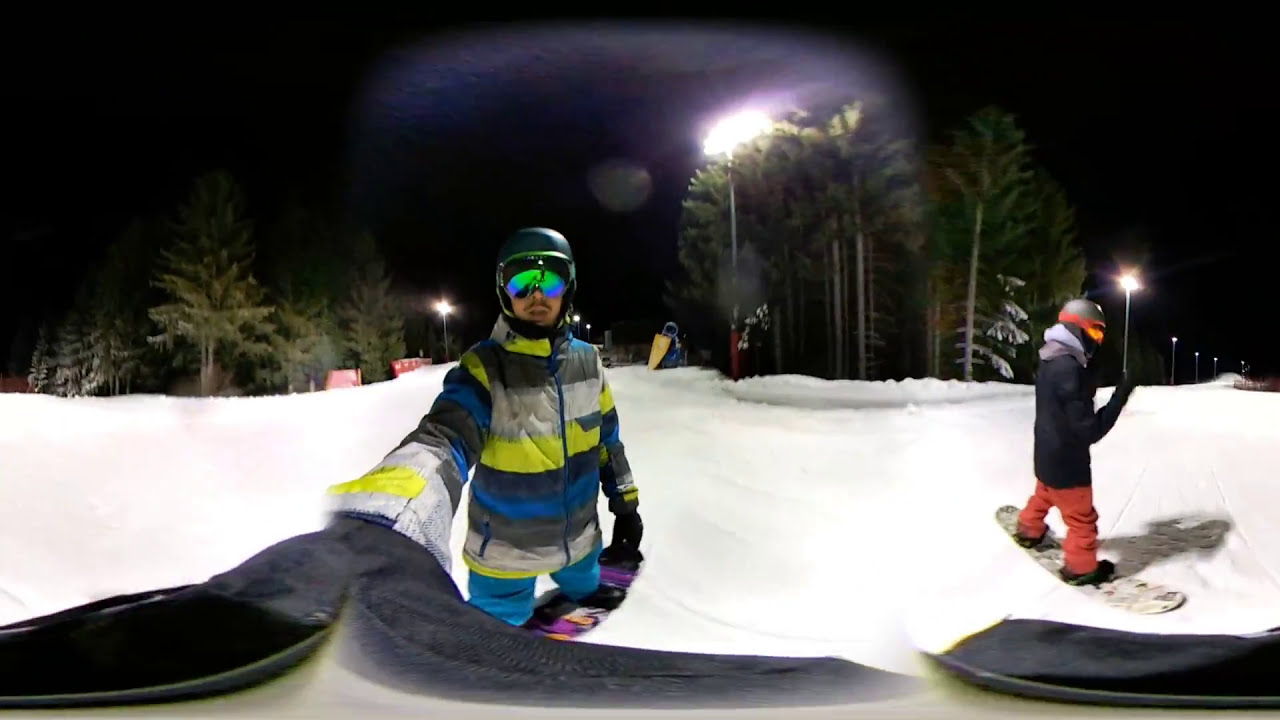In a striking nighttime scene, two snowboarders pose for a selfie amidst a snowy landscape, their figures appearing slightly distorted by the wide-angle lens. The snowboarder taking the selfie stands prominently to the right, his right arm outstretched to hold the camera. He sports a colorful snowsuit with yellow, blue, gray, and white stripes, complemented by a helmet and glasses that cover his eyes. His mustached face beams with excitement. Beside him, the other snowboarder, dressed in reddish-orange pants, a black jacket, and a helmet, looks downward, adjusting his stance on his snowboard. Behind them, trees stand stark against the black sky, with a faint moon visible amidst a purplish hue from ambient lighting. The entire scene is bathed in the soft glow of nighttime light, reflecting off the snow that blankets the ground.